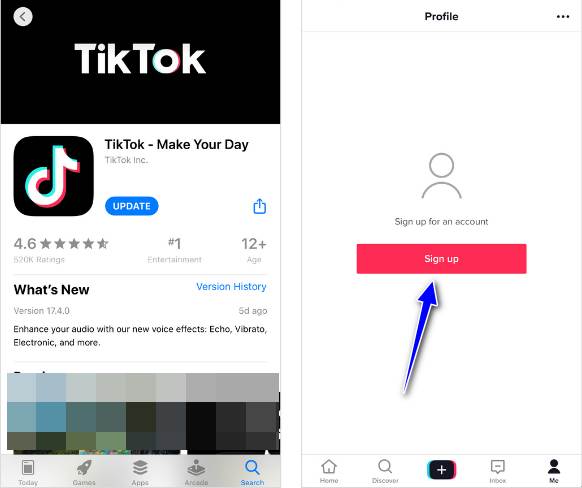A detailed screenshot of the TikTok app update screen is displayed on the left side. The header area prominently features the TikTok logo in white letters against a black background. Underneath, the phrase "TikTok: Make Your Day" is visible next to a black square featuring a white "like" symbol. Further below, it reads "TikTok Inc." followed by an ellipsis and the word "update" next to a blue square with an upwards arrow.

The app has a rating of 4.6 stars, as indicated by star icons and the text "570K ratings." It is mentioned as the "#1 in Entertainment" and carries a "12+ age rating." Directly under, there's a section titled "What's New" and "Version History," where it highlights the latest version, "17.4.0," which was updated 5 days ago. The update details include enhancements to audio features with new voice effects like Echo, Vibrato, and Electronic, among others.

The image contains a pixelated and blurred section obscuring part of the app screen. At the top right, there are tabs labeled "Today," "Games," "Apps," "Arcade," and "Search." To the far right, users are prompted to sign up for an account, represented by a black silhouette and a red button with the text "Sign Up" in white, accompanied by a blue arrow.

At the bottom navigation bar, icons include "Home," "Discover," a black box with a white plus sign, "Inbox" with a black chat box, and "Me" represented by a black silhouette of a person.